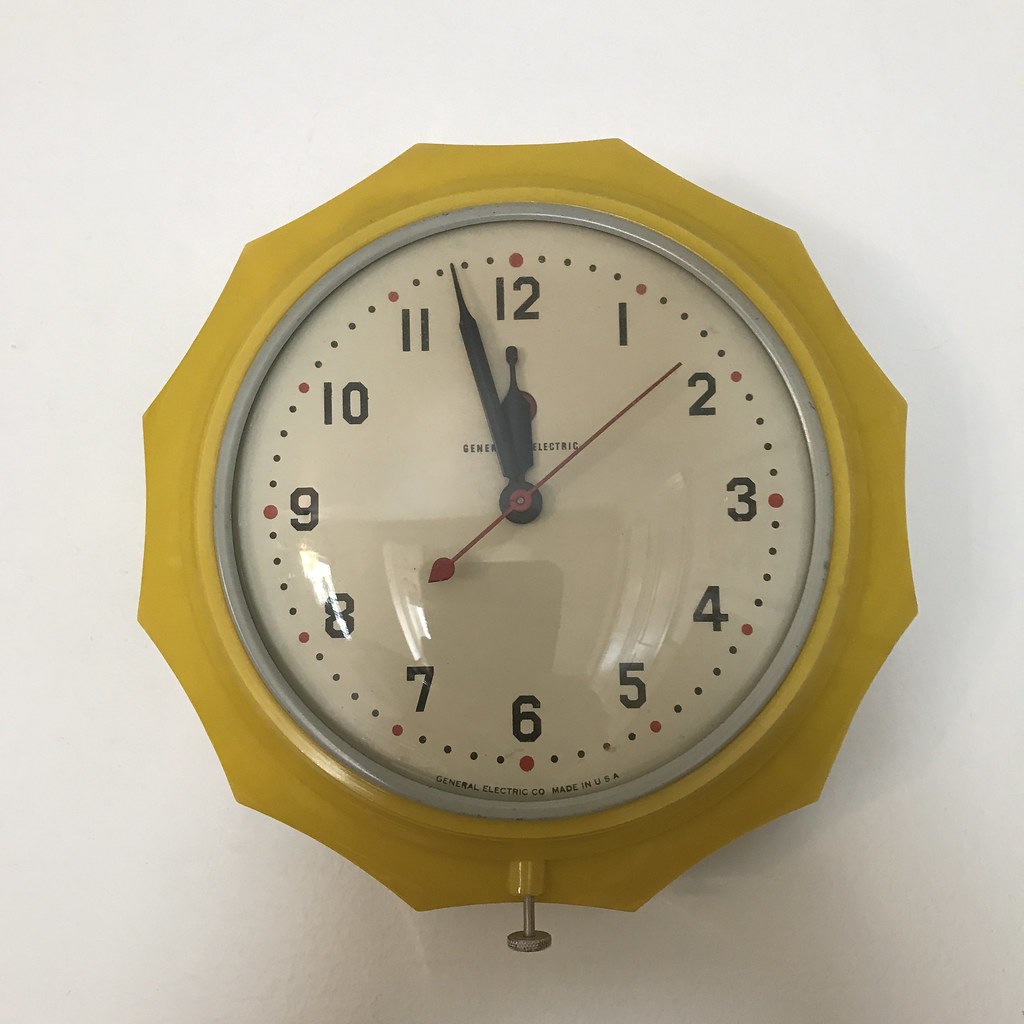This image features a wall-mounted clock against an off-white background with some gray shadowing at the bottom. The clock is centrally positioned and boasts a unique mustard-yellow frame with a dodecagon shape, reminiscent of a star or flower due to its semi-circular indented edges. The clock’s inner bezel is silver, complementing the white face adorned with black block numbers. Each hour is marked with small red dots, with larger red circles at 3, 6, 9, and 12 o’clock positions. The clock has black hour and minute hands, a red second hand, and an inscription below the hands that reads "General Electric Company made in USA." The frame includes a wind-up screw at the bottom in silver. The time displayed is approximately 11:58.